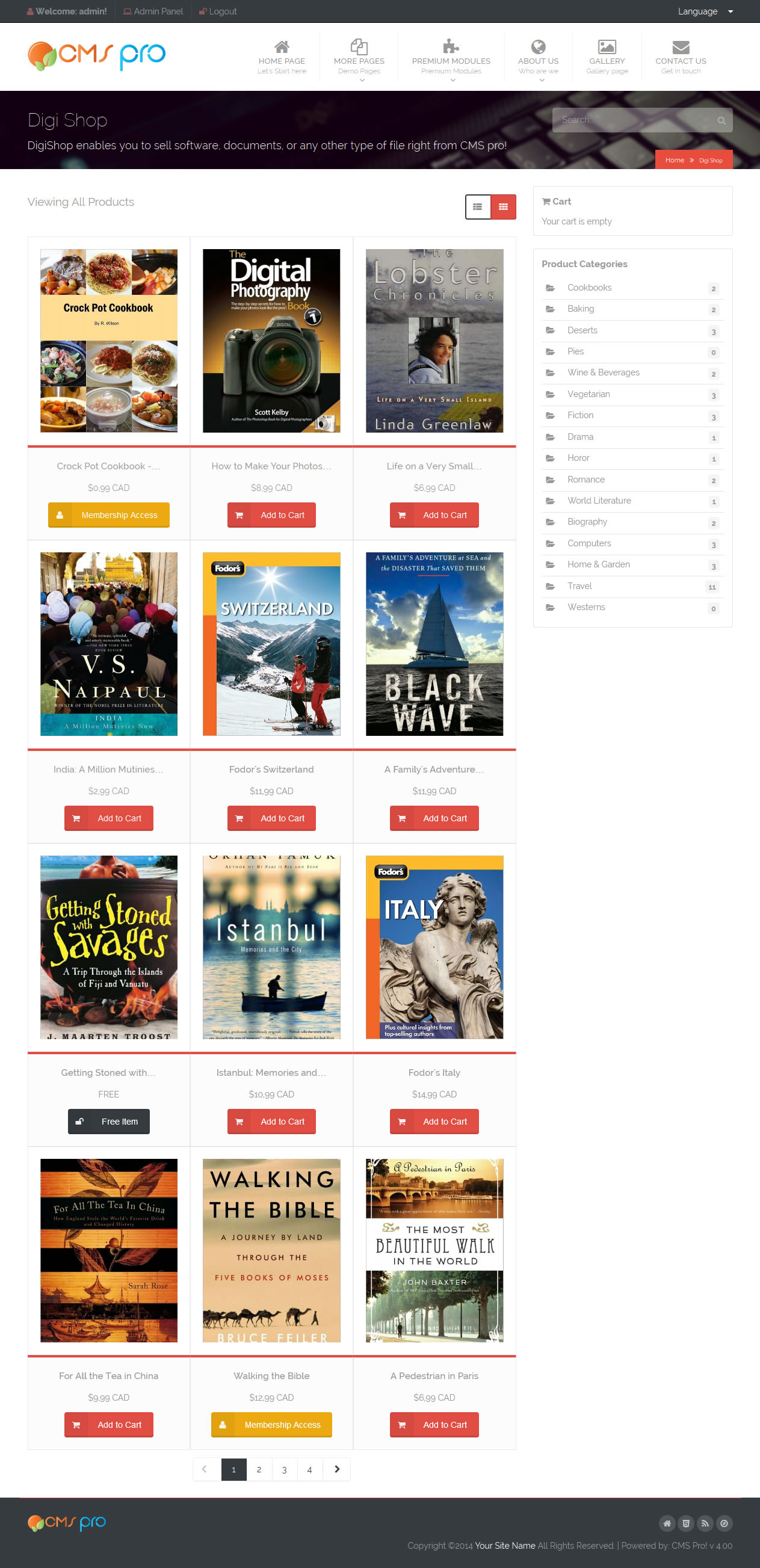This is a cropped screenshot of the CMS Pro desktop website. The image captures the interface, highlighting its organized layout and key elements. At the top, a white header spans the width of the page, displaying the CMS Pro logo on the left. The logo features an upside-down orange emblem with leaves pointing downward, followed by the letters "CM" in large orange font, a curved, slanted "S," and the word "PRO" in lowercase, large blue letters.

To the right of the logo, there is a navigation bar with categories listed horizontally: Home Page, More Pages, Plugins, About Us, Gallery, and Contact Us. Below this header, a black banner stretches across the top of the page. On the left side of this banner, smaller gray text reads "DigiShop," accompanied by a short description underneath. Toward the right of the banner, a search bar is prominently positioned at the top. Below the search bar and angled towards the bottom right of the black banner is a striking red button with white text.

The body of the page is white, featuring a vertical list of product thumbnails extending down the page. Each thumbnail displays a photo at the top, with the product title centered below in gray text. The price is aligned below the title, also in gray, and beneath that is an "Add to Cart" button.

This clear and organized layout facilitates easy navigation and user interaction, making it efficient for users to browse products and access various sections of the website.